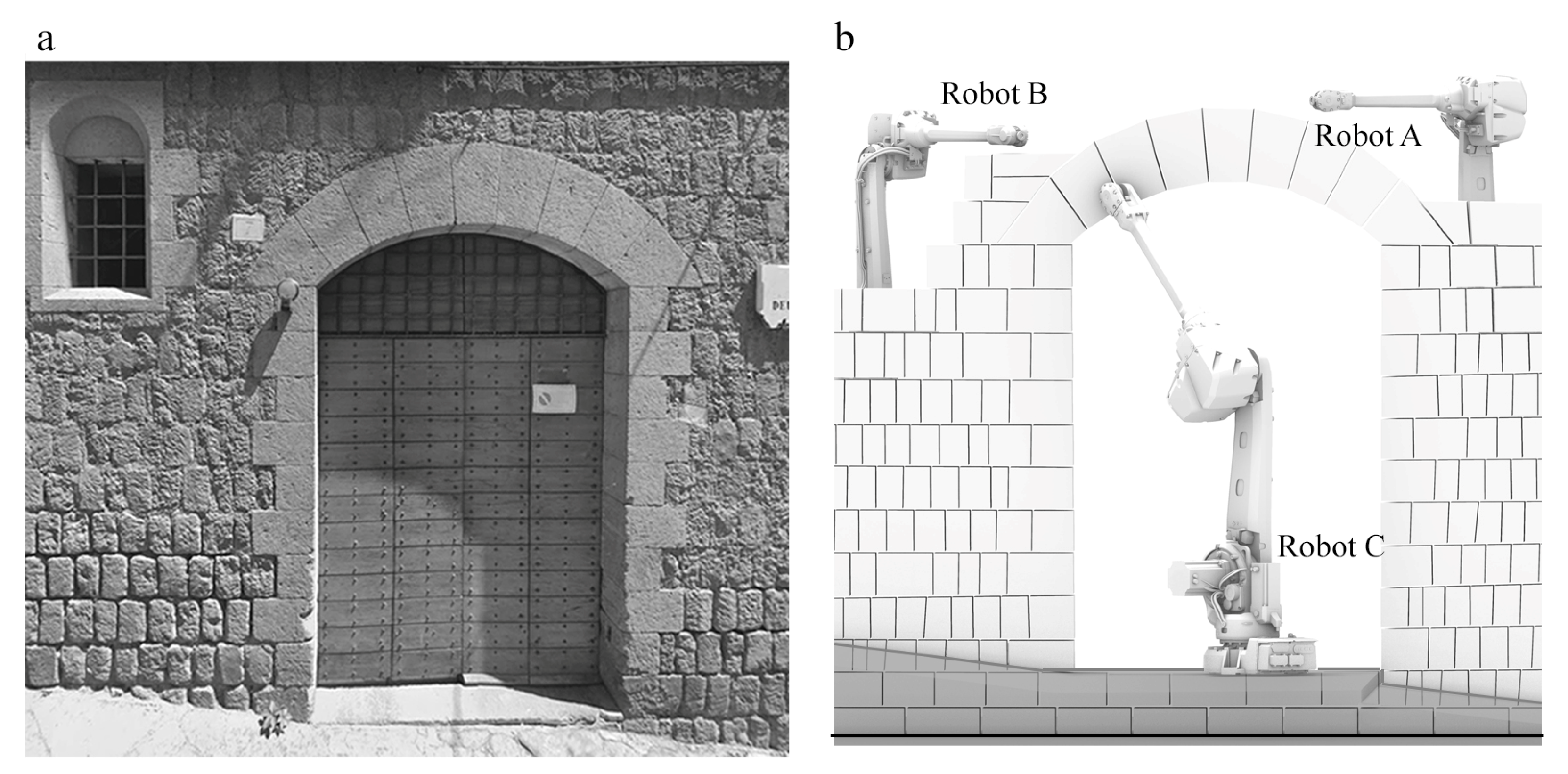The black and white image is divided into two labeled sections, "A" on the left and "B" on the right. The left side (A) features a close-up of a stone-like building's door, characterized by its arched stone seal and a small window situated at the top left. The door is visibly shut and designed to open outward from the center.

On the right side (B), the image depicts the same stone-like structure and door. However, this scene includes three small white robots. Two of these robots are positioned above the door, one on the left and one on the right. The third robot is located within the hollow area of the door. The robots are labeled respectively as Robot A, Robot B, and Robot C.